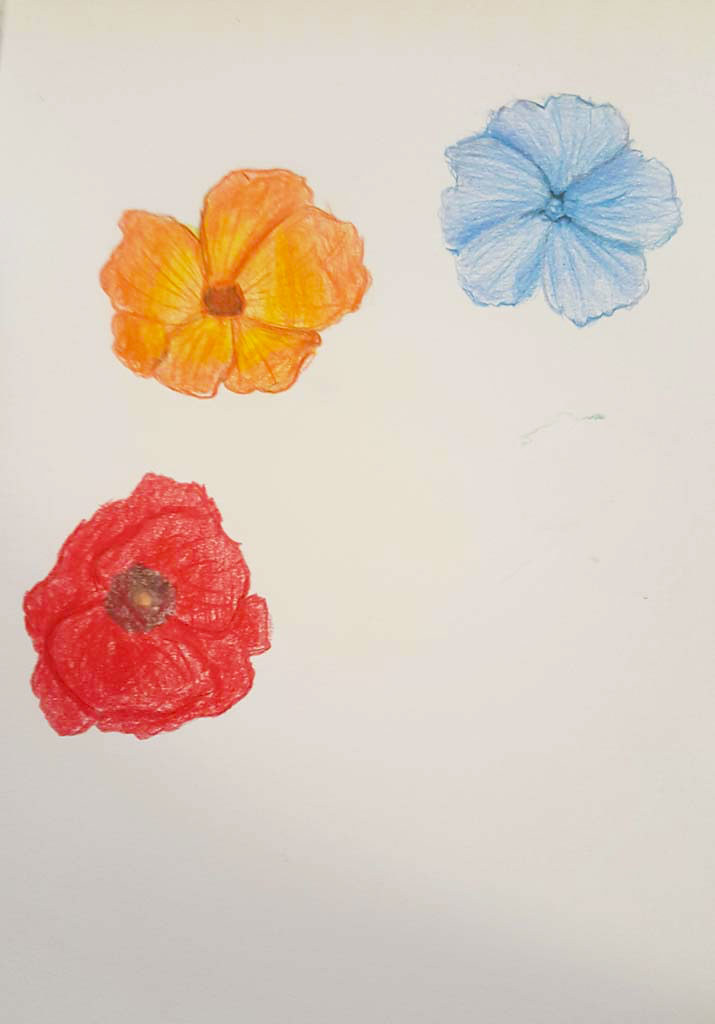This is a vertically oriented drawing on a white piece of paper. The artwork features three distinct, vividly colored flowers. Starting from the left, there is a red flower with a brownish-yellow center, displaying two prominent petals. Above this, positioned slightly higher, is a yellow flower with a similar brown center, from which vertical lines radiate towards the outer edges of the petals, adding depth and texture. To the right of the yellow flower, situated in the top right corner, is a blue flower with five petals and a blue circular center, also detailed with vertical lines emanating from the center. The careful use of colors and detailed petal work bring these flowers to life on the page.